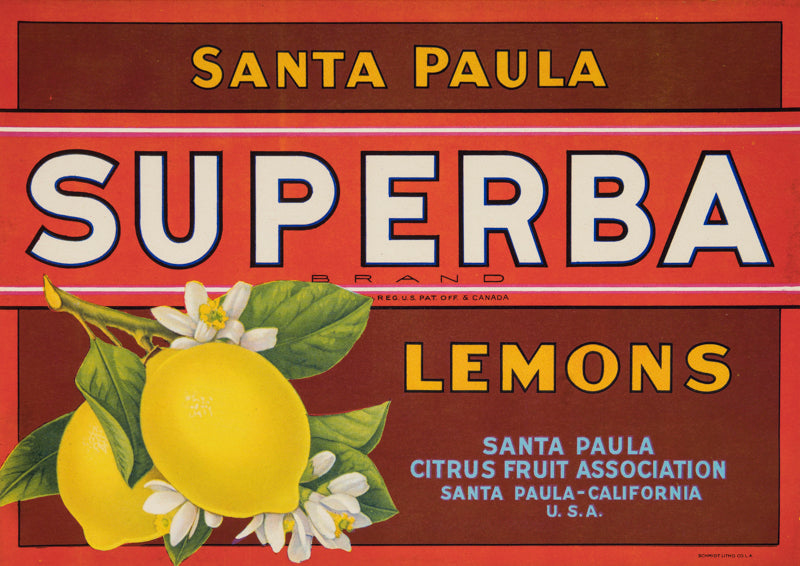This vibrant poster advertising lemons from the Santa Paula Citrus Fruit Association features a dynamic maroon background with a lighter maroon border. At the top of the poster, "Santa Paula" is prominently displayed in bold yellow text with a black outline. Below this, a large light maroon banner showcases the word "Superba" in white letters with a black outline, along with smaller text indicating "Brand." On the left side of the poster, there's an artistic rendering of two ripe lemons hanging from a branch, accompanied by white blossoms and lush green leaves. Below the illustration, the word "lemons" appears in the same bold yellow text. At the bottom right, smaller blue text reads "Santa Paula Citrus Fruit Association, Santa Paula, California, USA." The overall design is an eye-catching blend of bright colors and detailed illustrations, giving a modern and computerized feel to the classic fruit advertisement.